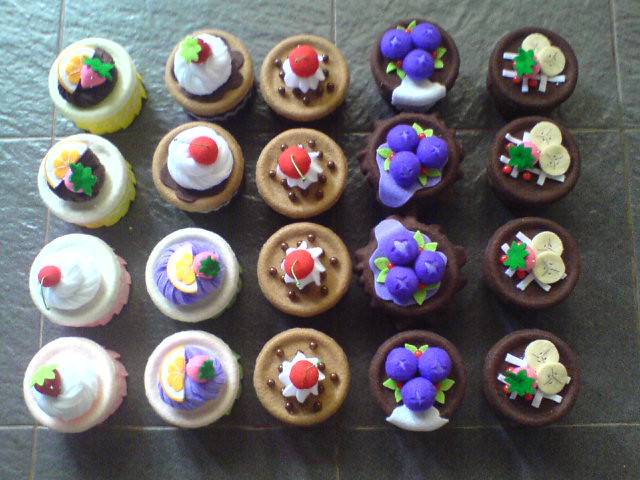The image showcases a top-down view of twenty intricately decorated cupcakes arranged in four rows and five columns, resting on a square-tiled green-gray surface. Each cupcake boasts unique decorations and vibrant colors, enhancing their visual appeal. The far-right column features brown cupcakes adorned with two white circles and a pinkish fruit resembling strawberry, while the adjacent column highlights chocolate-topped treats with three purple, blueberry-like circles. Moving leftward, the middle column contains lighter brown cupcakes decorated with white and red circular embellishments. The leftmost cupcakes present a diverse array, including a white cupcake with an orange slice, another light brown one with a red circle, a yellow cupcake with white icing reminiscent of orange slices, and a pink-topped one with red circles. Each cupcake's decorative elements, from mounds of whipped cream to simulated fruits like cherries, strawberries, and bananas, add to the overall charm and sophistication of the display.